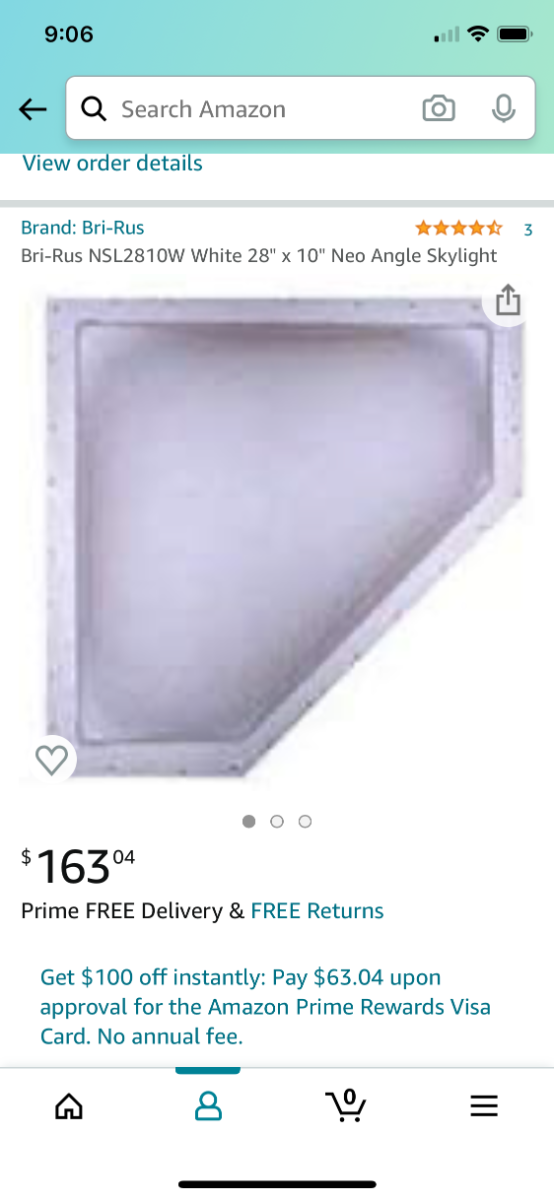The screenshot captures a phone display at 9:06 PM, showing full battery but minimal cellular reception with just one bar. However, the device has internet connectivity, as evidenced by an open Amazon search bar. Below the search bar, there's an option to view order details for a product from the brand Brie Russ. The item is a 28-inch by 10-inch neo-angle skylight, which appears to have gone through a peculiar design choice—it is neither a perfect rectangle nor a triangle but rather a unique shape created by skewing the lines of a rectangle. The product listing shows it costs $163.04, with options for free delivery and free returns. Additionally, there's a promotion for the Amazon Prime Rewards Visa card, offering a $100 discount on approval, reducing the cost to $63.04. The card boasts no annual fee, encouraging potential buyers to consider financing.